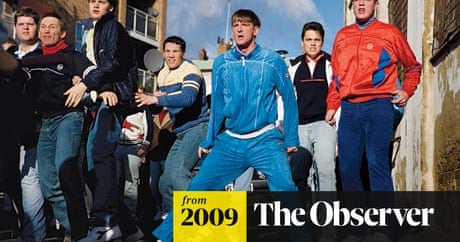The photograph from The Observer, dated 2009, captures a tense moment outdoors under a blue sky scattered with a few clouds. In what appears to be an alley flanked by concrete buildings—some slightly crumbling—stand a group of young men, all seemingly prepared for confrontation. The scene is accentuated by an old photo feel, with a yellow rectangle containing black text stating "From 2009" and a black rectangle with white text that reads "The Observer" at the bottom right corner.

Amidst the group, the individual in the center is particularly striking, dressed in a distinct blue sweatsuit. To his right, a man sports a red jacket paired with blue pants, contrasting with others who mostly wear blue jeans and various jackets. Specifically noted are a man in a white and blue shirt with blue jeans, another in a black jacket with blue jeans, and one in a black shirt featuring a white stripe, a red turtleneck underneath, and blue jeans. The diverse attire—ranging from jumpers to sweatshirts and jackets—complements the charged atmosphere as they all look off into the distance, seemingly amped up and ready for a potential altercation. The image's setting and the men's stances collectively evoke a sense of impending conflict.